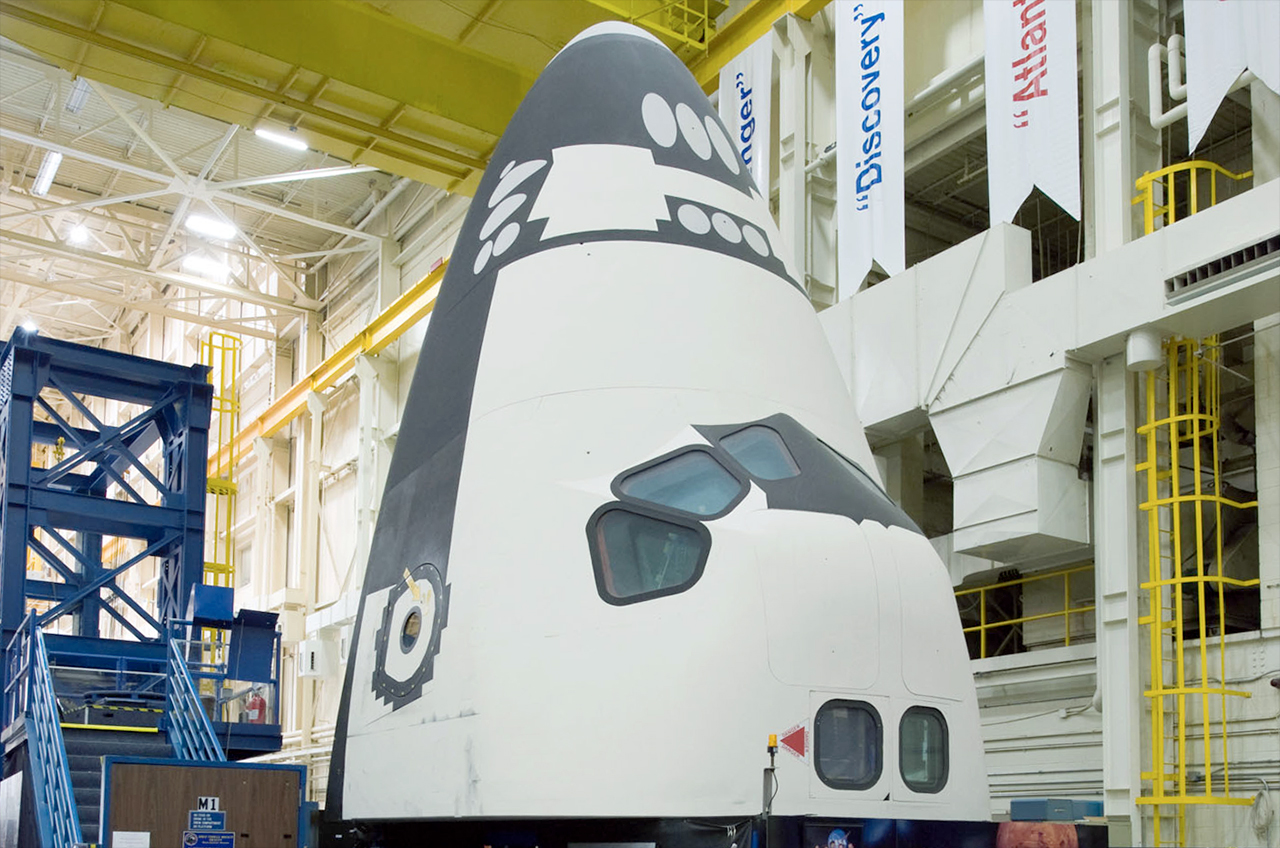This detailed image showcases the nose section of a NASA space shuttle on display at a museum, likely NASA's Space Center. The shuttle's nose is a white and gray cone, decorated with black trim and white spots, and is pointed upwards. Prominently featured are three polygonal windows at the front and two square windows on the top. A set of blue metal stairs to the left provides access, possibly for a closer view or entry into the shuttle. The backdrop reveals a large, industrial-style warehouse with steel support beams, yellow bars running between floors, and factory lights overhead. Several banners are hanging in the background, including ones labeled "Discovery," "Atlantis" (partially cut off), and possibly "Voyager.”